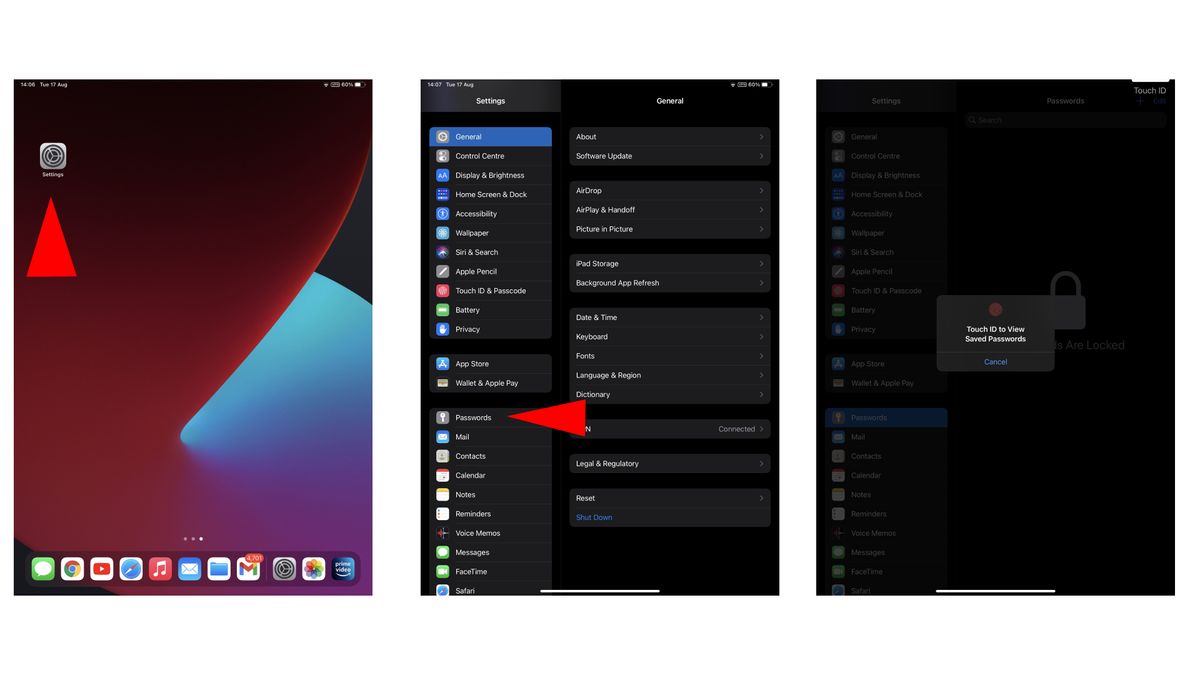This image is a landscape-oriented, three-column collage of screenshots from a smartphone. 

**First Column:**  
The image on the left displays the home screen of a smartphone, filled with various app icons. A prominent red arrow on the left side of the screen points upwards to an icon labeled "Settings." The background is an abstract blend of red and light blue circles. Apps visible at the bottom include icons for Messaging, Google, YouTube, a blue music app, an envelope icon (likely email), a calendar app, Google Photos, Prime Video, and another settings icon.

**Second Column:**  
The middle screenshot captures the Settings menu on the smartphone. A red triangle directs attention to the "Passwords" option. The menu includes sections like "Control Center," "Display & Brightness," "Home Screen," "Accessibility," "Wallpaper," "Siri & Search," "Touch ID & Passcode," "Battery," "Privacy," "App Store," "Wallet & Apple Pay," "Passwords," "Mail," "Contacts," "Calendar," "Notes," "Reminders," "Voice Memos," "Messages," and "FaceTime." Under the "General" heading, the options listed are "About," "Software Update," and "AirDrop."

**Third Column:**  
The screenshot on the right is darker, focusing on the "Touch ID to View Saved Passwords" prompt. In the middle of this screen is a distinct shape with a handle-like extension on the right side and a small red dot, resembling a fingerprint scanner. The "Cancel" option is mentioned as an alternative action. 

Overall, this series of images illustrates the steps for navigating through a smartphone's settings to access saved passwords using Touch ID.